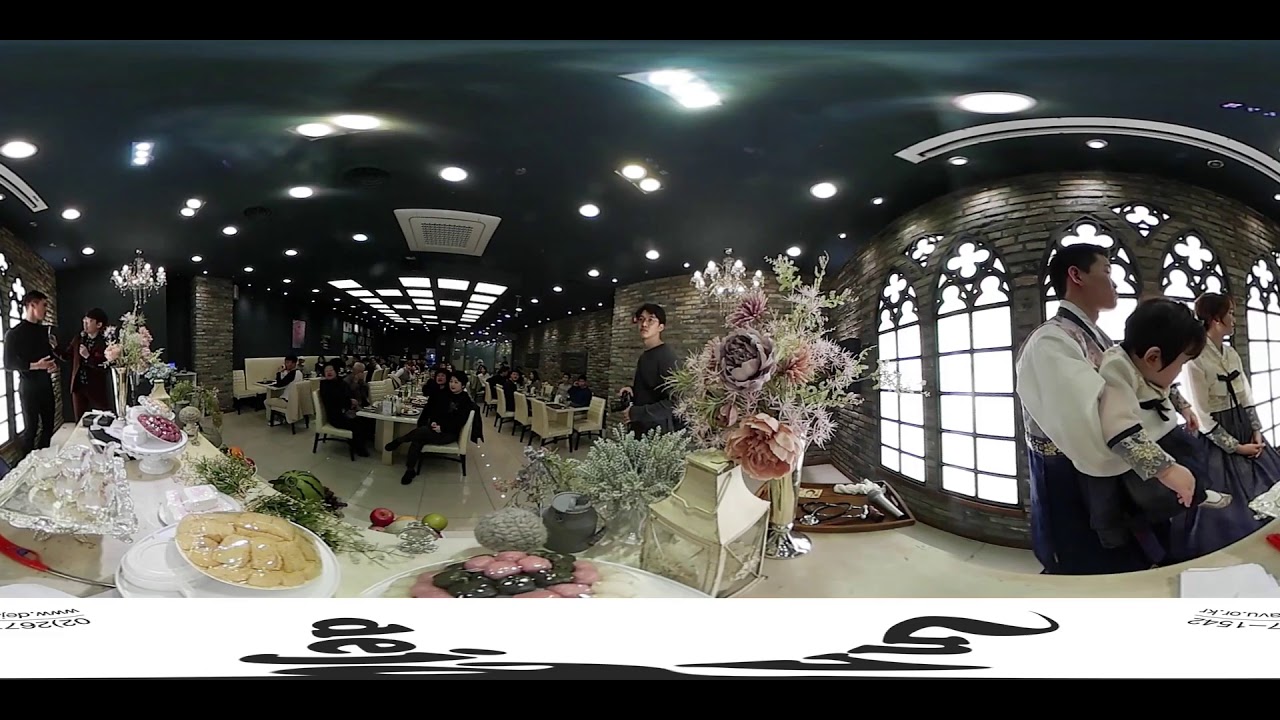The image captures a vibrant wedding reception scene, possibly an Asian wedding, characterized by its lively and celebratory atmosphere. Central to the image is a long, white table laden with an array of food, including an assortment of desserts and brightly colored flowers in square vases. The setting is adorned with numerous lights and chandeliers hanging from the ceiling, bathing the room in a festive glow. Rows of white-clad tables and chairs extend into the background, flanked by guests primarily dressed in formal black suits, although some individuals are wearing white outfits and ceremonial attire. To the right, a man in a white uniform apron lifts a child by the stomach, while another woman stands beside them, presumably part of the serving staff. The surrounding environment includes paneled windows and brick walls, adding to the event's elegant backdrop.